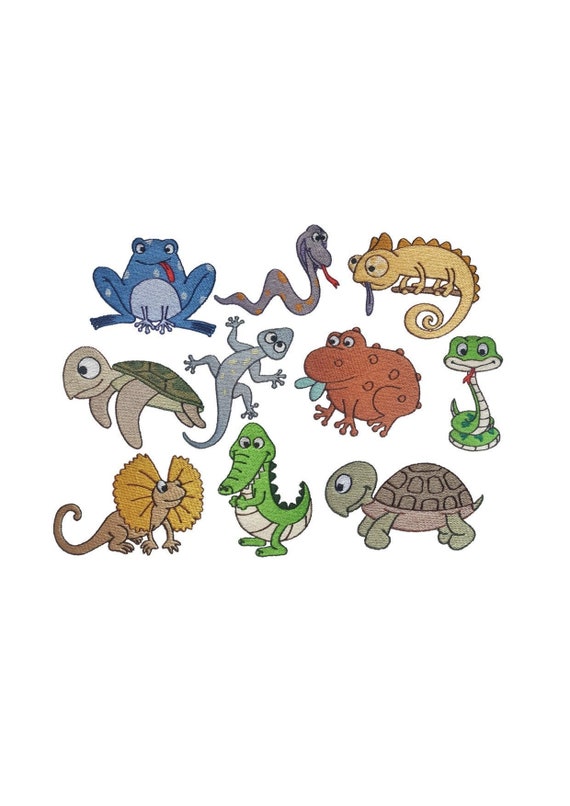The image features ten colorful, cartoon-style drawings of various small animals and amphibians, all set against a plain white background without any borders. The illustrations include a blue frog with its red tongue playfully sticking out, a gray snake curled up with its tongue extended, a typical green turtle, and a green alligator. There is also a green and cream-colored snake poised to strike, a lizard adorned with flaps on the side of its head, and a sea turtle. Additionally, the set showcases a comical big bullfrog with warts, a dynamic green tortoise, a gray chameleon at the top, jaunty and ready, and a tiny red creature that resembles a plump, fat animal. Each character is drawn with amusing expressions, characterized by funny eyes and engaging faces, making the entire ensemble appear particularly charming and amusing.